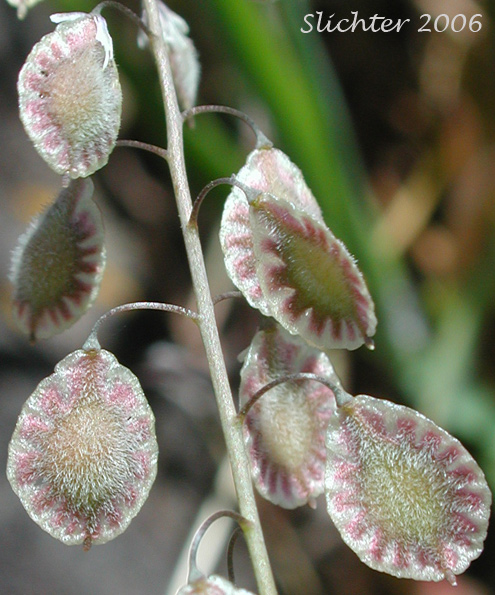In this high-definition macro photograph taken by Schlichter in 2006, a visually stunning plant is showcased with remarkable clarity. The central subject features a plant stem adorned with several teardrop or oval-shaped leaves, each exhibiting a unique coloration. The leaves are predominantly white with pinkish dots, featuring edges trimmed in white. The center of the leaves displays shades of yellow and brown, giving them a slightly translucent appearance. These leaves appear to be covered in minute white hairs, contributing to a furry texture. The stem itself is light green with hints of whitish coloration and has a subtle shine, indicating a textured surface.

The background is artistically blurred using a bokeh effect, drawing attention to the plant while softly hinting at the greenery and other plants behind it. This soft-focused background includes blurred blades of dark green grass and other indistinct plant forms, suggesting a natural setting. The subdued lighting in the background likely stems from the use of artificial light focused on the plant, enhancing its vivid and intricate details against the softer backdrop.